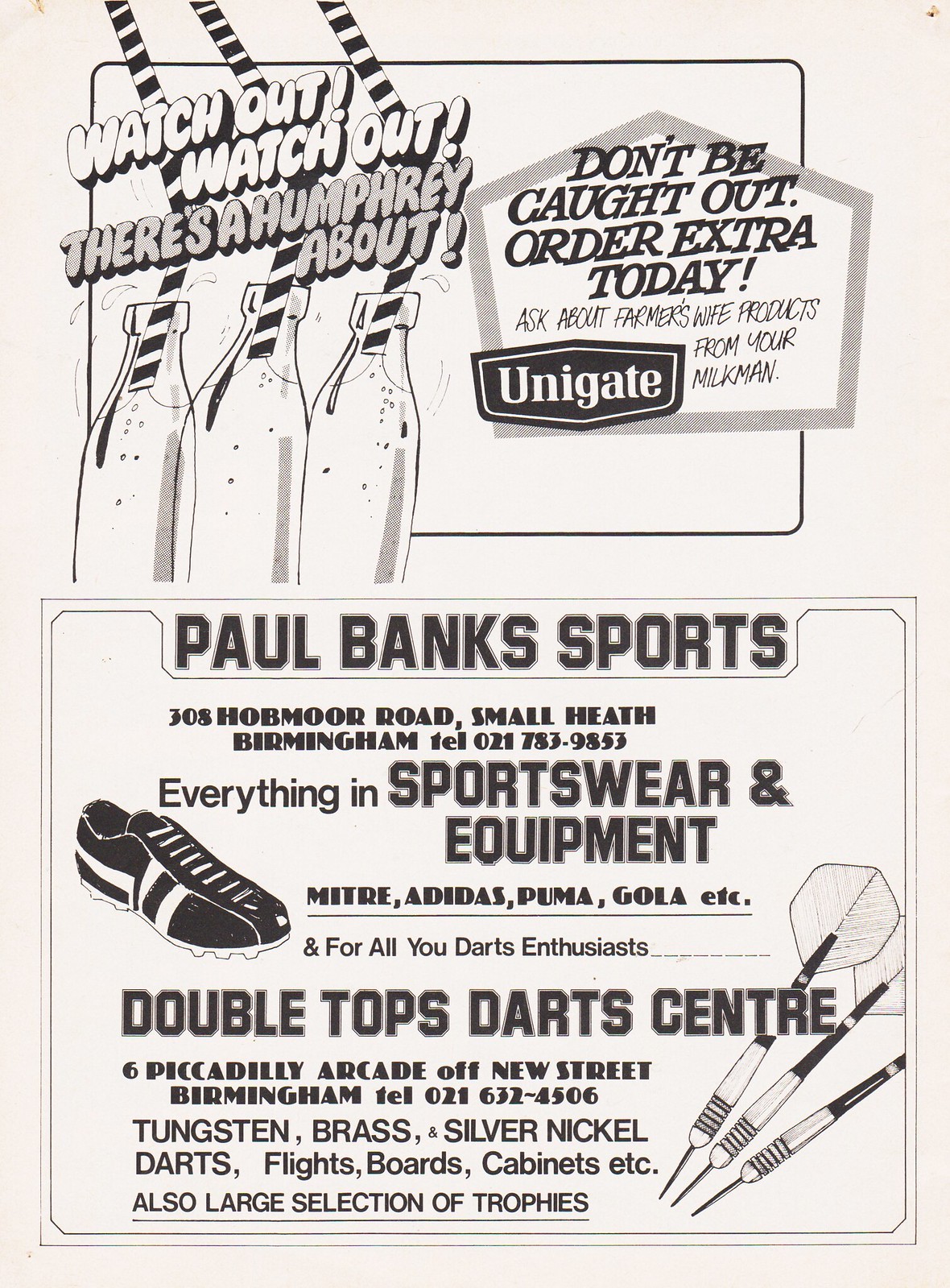The image is a tall, rectangular flyer with an off-white background divided into two main sections, featuring a vintage theme. At the top, the flyer showcases an advertisement with three illustrated soda bottles, each adorned with black and white striped straws. Above these bottles, in white bubble letters, are the words "Watch out, watch out," followed by "there's a Humphrey about" in gray bubble letters. To the right, within a gray pentagon shape, it urgently advises, "Don't be caught out, order extra today. Ask about Farmer's Wife products from your milkman," underlining Unigate's promotion.

Below this ad, the flyer transitions into a bold sportswear advertisement for Paul Banks Sports, located at 308 Hobmore Road, Small Heath, Birmingham. It highlights everything from major brands like Mitre, Adidas, Puma, and Gola. Additionally, it caters to darts enthusiasts under the banner "Double Tops Darts Center" at 6 Piccadilly Arcade, off New Street, Birmingham. The ad provides intricate details, listing products such as tungsten, brass, silver-nickel darts, flights, boards, cabinets, and numerous trophies, accompanied by corresponding imagery—a soccer cleat and darts. The contact numbers, 021-783-9853 and 021-632-4506, are also included for prospective customers.